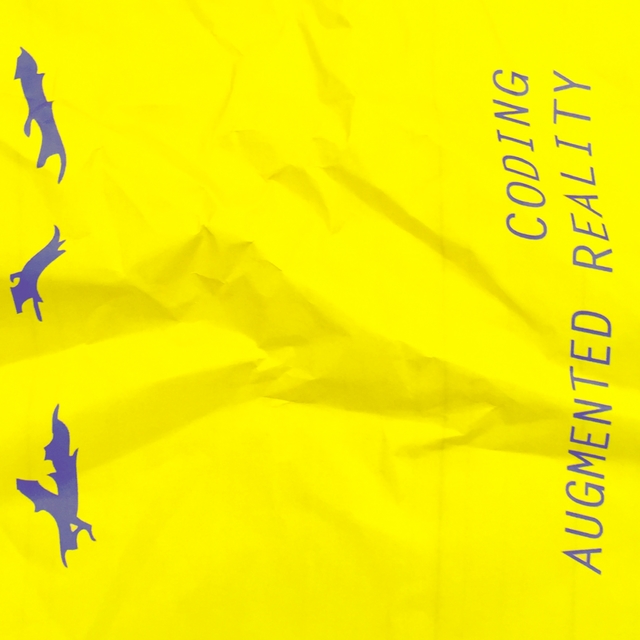The image depicts a crumpled yet spread-out piece of yellow paper, its surface covered in numerous wrinkles and crinkles from having been previously crumpled up. On the left side, the paper features three abstract, fluid, and wavy shapes in a bluish-purple hue, each with numerous sharp, pointy edges. These shapes are arranged in a column-like manner with spaces in between; the top resembles curled purple ribbon, the middle morphs into a claw-like design, and the bottom is V-shaped. On the right side of the paper, at a vertical and sideways angle, is the text "Coding Augmented Reality" written in blue or purple, all capitalized, creating a striking contrast against the yellow background. These elements together give the image the style of a poster adorned with abstract illustrations and bold typography.